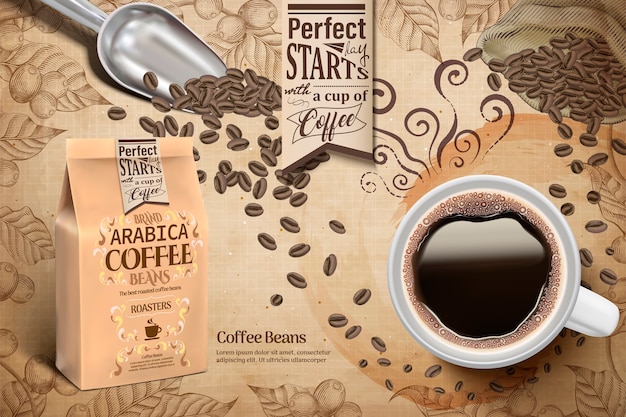In this detailed advertisement image for coffee, we see a meticulously crafted layout featuring a blend of photographic and illustrated elements. The background is a beige, botanical illustration style canvas adorned with detailed drawings of coffee plants, leaves, and coffee cherries. Central to the composition is an overhead view of a steaming cup of coffee in a white mug, realistically rendered with bubbles around the rim, enhancing the fresh, inviting appeal of the beverage.

To the left, an illustration of a brown coffee bag with a slightly reddish hue is prominently displayed. The bag is labeled with "Brand Arabica Coffee Beans Roasters" and a detailed illustration of a coffee cup. The top of the bag is folded over, suggesting it has been opened, with some beans spilling out.

Dominating the upper right section, a metallic coffee scoop filled with realistically illustrated roasted coffee beans directs a cascade of beans downward, guiding the viewer's eye toward the cup of coffee. The scoop's handle points toward the top left, contrasting with the carefully illustrated beans that tumble towards the main coffee cup.

A ribbon-shaped banner across the top center reads, "The Perfect Day Starts With a Cup of Coffee," effectively drawing attention and providing a welcoming message. Additionally, stylized, brown curlicue illustrations of steam rise from the coffee cup, adding a whimsical touch that compliments the realistic details. The intricate artwork and realistic depiction combine to create a visually engaging and appetizing presentation, perfectly encapsulating the essence of a delightful coffee experience.